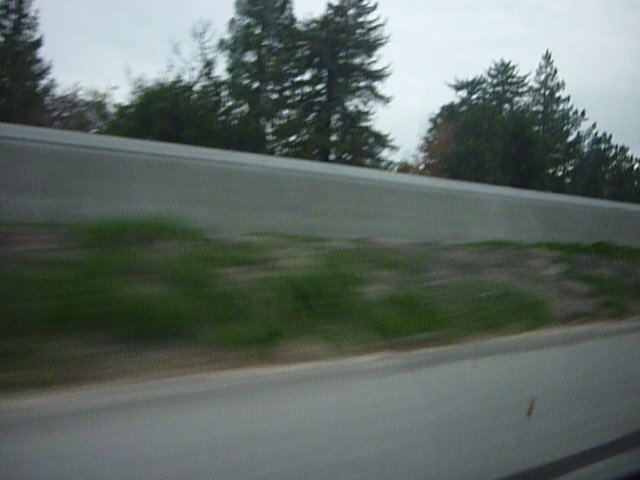The image is a blurry scene, seemingly captured from a moving car. In the background, there are tall trees silhouetted against a gray, overcast sky. A prominent white strip, possibly a cloud or a light-colored structure, cuts across the sky. Below the trees, there is a mix of green grass and patches of bare, brown dirt, suggesting an area that is not fully vegetated. Further down, there appears to be a large, beige structure that looks like a wall or barrier, which contributes to the image's odd and disjointed appearance due to the motion blur.